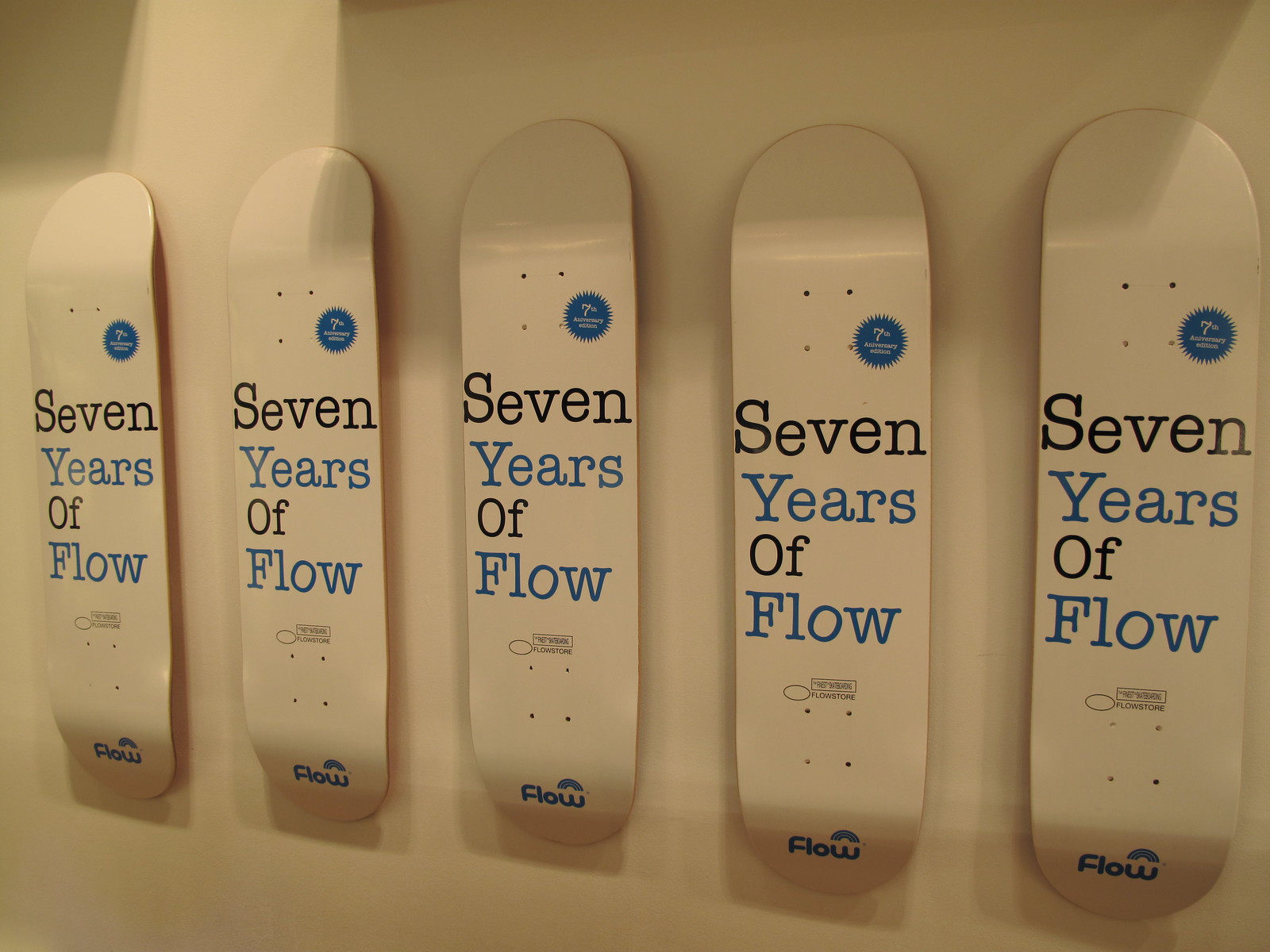The image depicts a set of five identical skateboard decks, mounted uniformly on a white wall in a vertically spaced arrangement. Each deck is white and prominently features a blue logo at the top, resembling a badge or stamp, indicating the company's seventh anniversary. Beneath this, in large alternating black and blue letters, is the text "seven years of flow" with each word on its own line. The bottom portion of each skateboard includes a logo of the company "Flow," featuring a distinctive blue and white water logo or rainbow above the letter "W." The boards are devoid of wheels and trucks, emphasizing their decorative or commemorative purpose, possibly displayed in a gallery or company office setting. The overall background is relatively dark, suggesting limited artificial lighting in the room where the photo was taken.